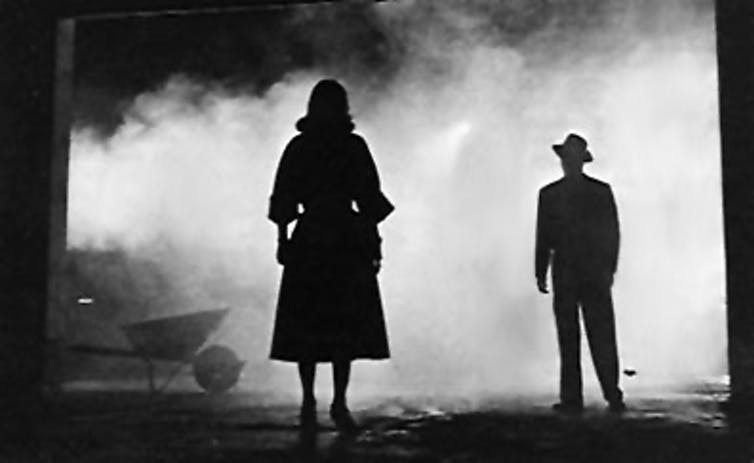In a striking black-and-white image enveloped in dusky fog that resembles white clouds, a man and a woman confront each other in the night, their forms reduced to silhouettes. The man, standing to the right, is sharply dressed in a suit and a classic hat from the 40s or 50s, with his arms calmly at his sides. Opposite him, to the left, the woman is clad in a long, flowing gown or overcoat that reaches her mid-calf and wears her dark hair cascading over her shoulders. This mysterious scene is set against an indistinct, dark background, possibly within a farmhouse or barn, heightening the cinematic suspense reminiscent of a still from an Alfred Hitchcock film or similar dark-themed movie. Adding to the vintage atmosphere, a wheelbarrow is positioned to the left of the frame, its handles and front wheel faintly visible through the dense fog. The interplay of light and shadow accentuates the tension and surprise of their confrontation, making their expressions indecipherable yet evocative in their enigmatic encounter.